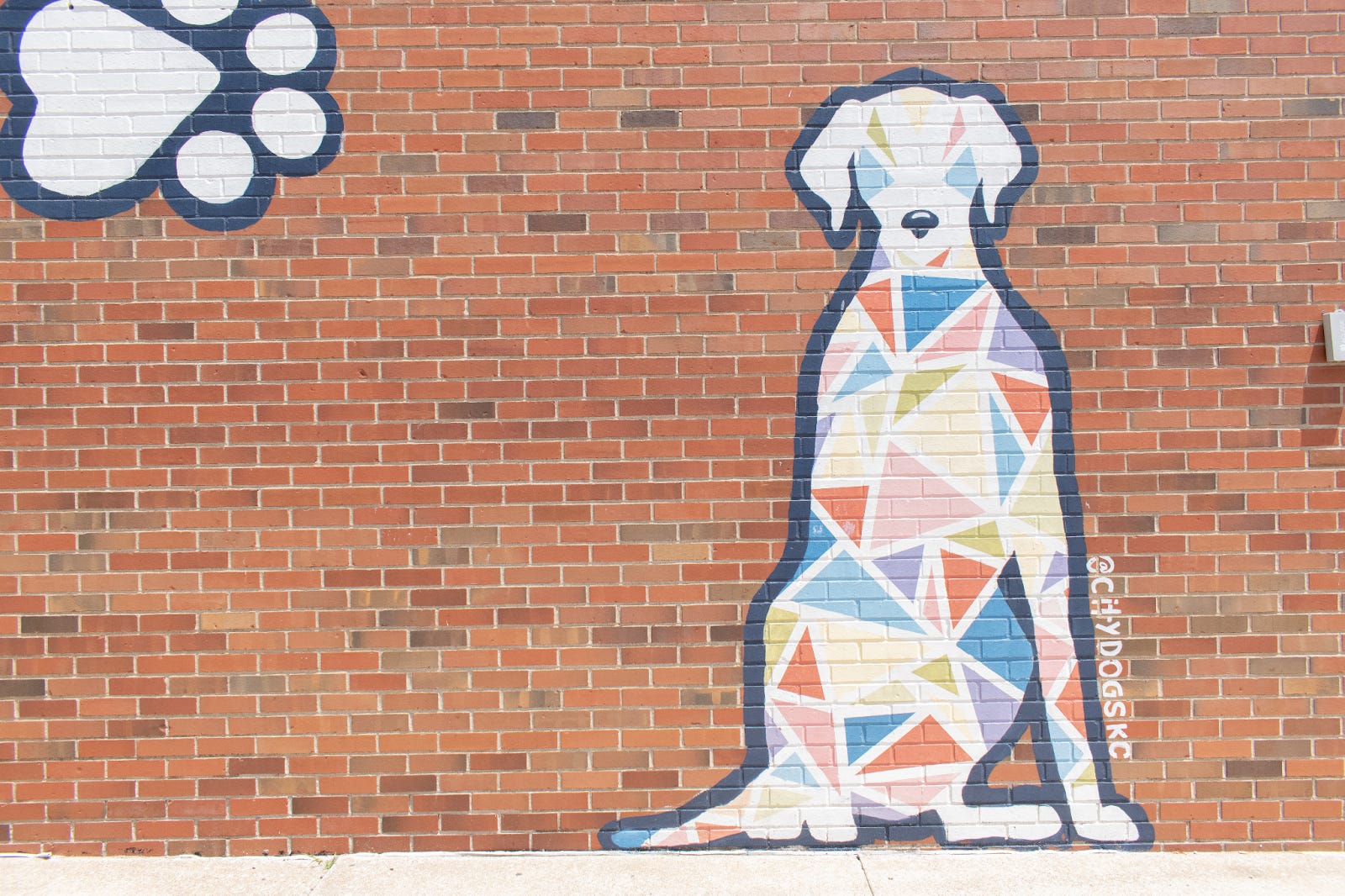The image captures a vibrant piece of graffiti art on a large red brick wall that extends from top to bottom and side to side. Off-center to the right, there is a detailed and colorful polyart painting of a seated dog, outlined in thick black paint. The dog faces forward with its black nose, ears perked and slightly drooping on either side. Its body is composed entirely of variously colored polygonal triangles in shades of light blue, red, pink, green, tan, orange, and white. The dog's visible foreleg extends downward, while its tail curves slightly to the left of its body. In an upper corner of the wall, there is a smaller depiction of a dog's paw print painted in white and outlined in black. The paw features a heart-shaped pad pointing to the right and three visible toe pads. Additional details include small, difficult-to-read white lettering near the right side of the dog that appears to say "copyright chydogs.kc." The artwork juxtaposes with the red brick canvas, featuring vivid colors and rich geometric patterns, giving a sense of organized chaos typical of commissioned street art.